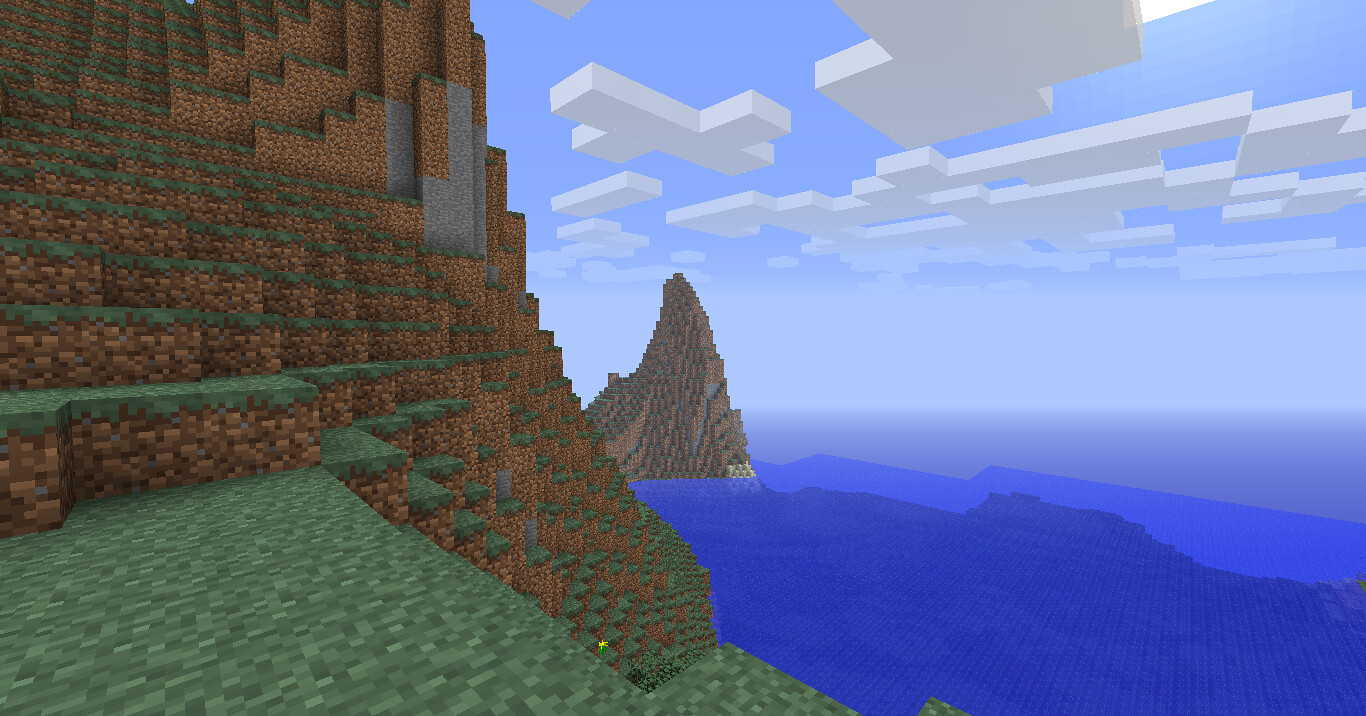This still image from a Minecraft game showcases a diverse landscape with pixelated charm. On the left, a mountain with brown and green hues rises steeply, embodying the characteristic blocky design of Minecraft terrain. To the right, an expansive ocean stretches out, its water transitioning from a dark blue in the foreground to lighter shades as it recedes into the horizon. Above, a splendid sky shifts from a vivid, darker blue at the top to a more subdued tone near the ocean's edge, dotted with light and dark gray clouds adding texture to the scene. In the far left-middle of the ocean, another mountain peak juts out, its rocky, brown prominence topped with patches of green, culminating in an impressively sharp point, all contributing to the depth and vibrancy of this virtual world.